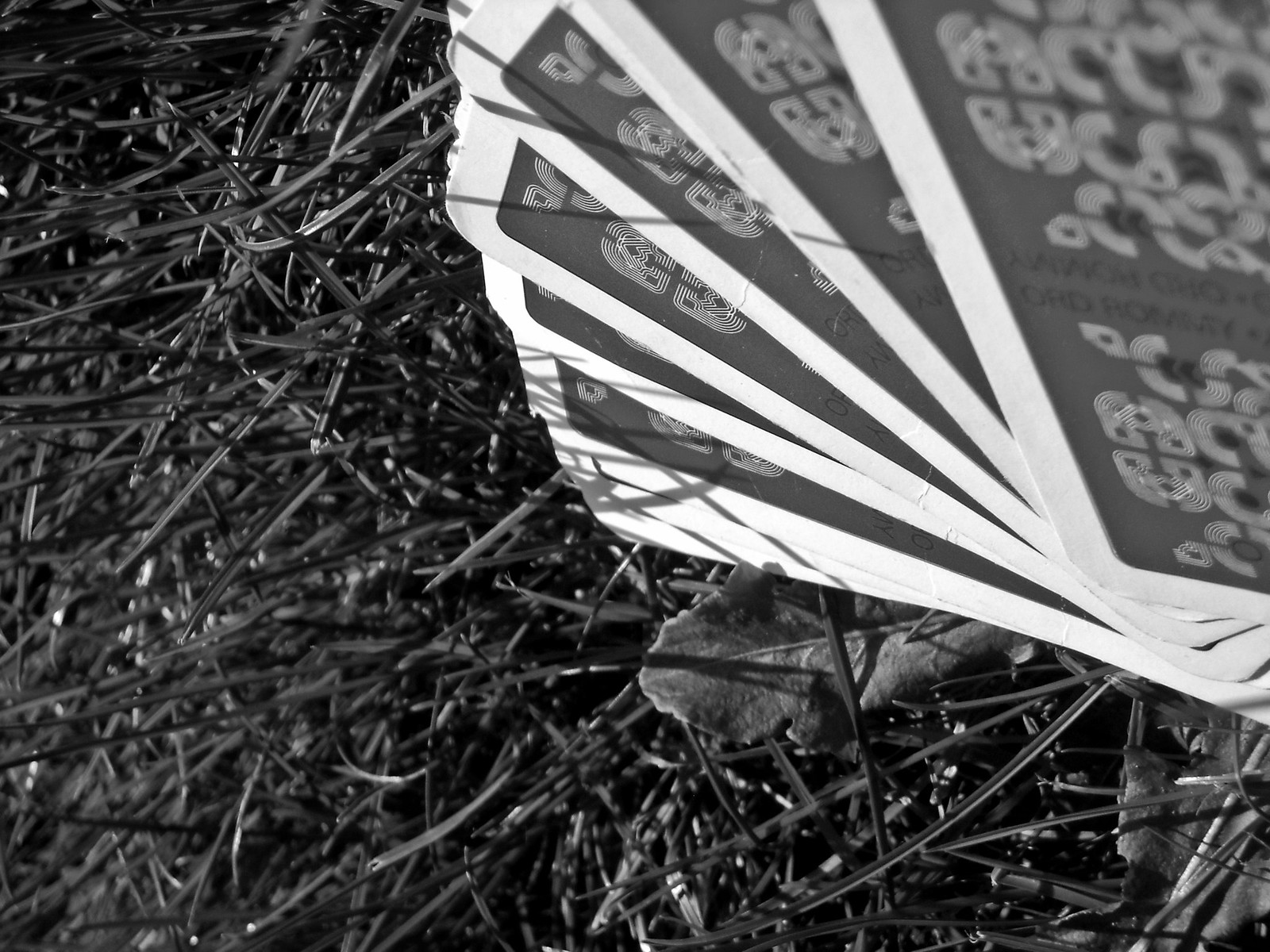The image showcases an outdoor, close-up shot of the ground. In the top right corner, several white-outlined cards are scattered. These cards feature intricate designs resembling hieroglyphs or textures that evoke images of worms and other organic shapes, though the details are difficult to discern. In the bottom left corner, lush green grass and scattered leaves are seen, contrasting with the predominantly black-and-white scene. The overall composition is a juxtaposition of natural elements with the mysterious cards. The text on the cards is in black, with gray designs and white outlines, adding to the enigmatic feel as the text remains largely unreadable.